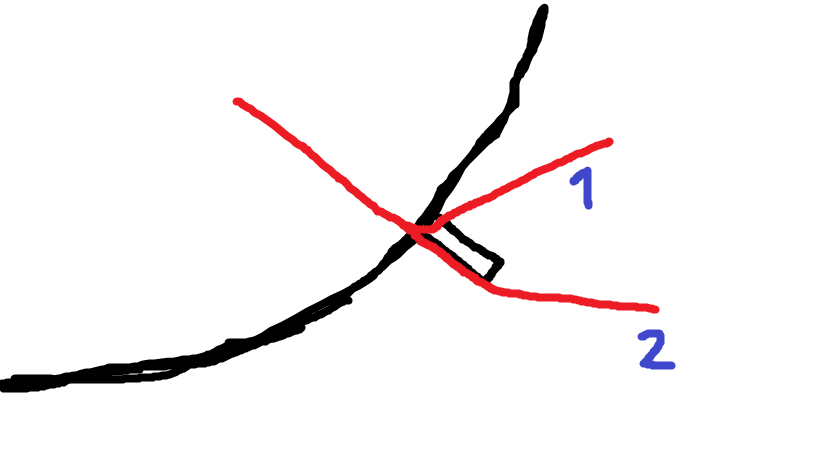The image appears to be a screenshot of a digitally created drawing in a basic graphic software, likely Microsoft Paint. The background is a solid, opaque white with hand-drawn, freeform lines. A slightly curved black line, reminiscent of a smile, extends from the bottom left towards the upper right corner of the image. Intersecting this curve, a black rectangular box is drawn around the midpoint, extending towards the bottom right. Above this setup, a red line forms a horizontal Y-shape lying on its side. The left branch of the Y is positioned above the intersection, while the right branch extends towards the bottom right of the image. Additionally, the branches of the Y are labeled with the numbers "1" and "2" in purple.